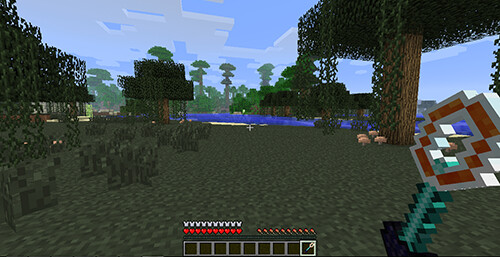The image depicts a scene from the video game "Minecraft," set in a virtual world. The bottom of the image features a dark green grassy area dotted with eight or nine short, round bushes on the left-hand side. Continuing up the left side towards the top left, there is an elevated wrought iron railing adorned with ivy that cascades over the open areas of the fence. 

In the center of the image, there's a structure resembling a treehouse, shrouded in hanging ivy, behind which stretches a royal blue body of water. On the right-hand side, more wrought iron railings are present, strung with ivy and supported by sturdy wooden square pillars holding up an overhead structure. The sky at the top of the image is a distinctive "Minecraft" blue, peppered with cuboid white clouds.

At the bottom center, the Minecraft interface elements are visible: numerous gray cubes with green centers, a series of red hearts indicating health or lives on the left, and what seems to be a red flower on the right. Additionally, a street-like area beneath a metal structure, possibly the underside of a bridge, can be seen, with several small gray characters scattered about. This blend of natural and constructed elements, along with the iconic health bar, affirms the unmistakable "Minecraft" aesthetic.